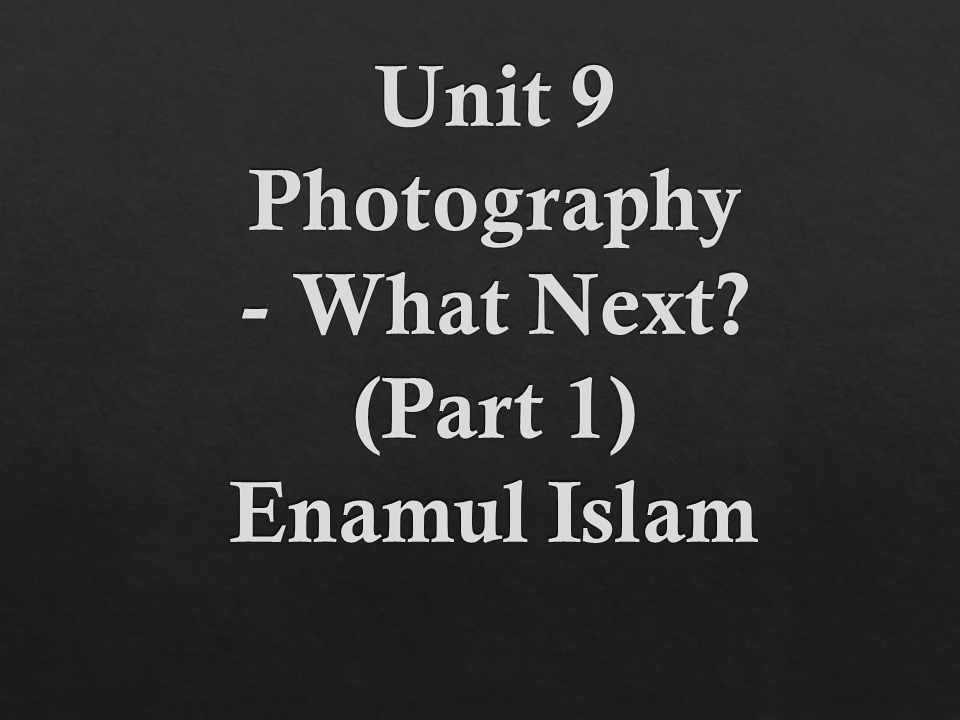This image features a sleek, minimalist design with white text against a solid black textured background. The text, centered closer to the top of the landscape-oriented rectangle, is written in a bold, serif font and is laid out in five lines: 

1. Unit 9
2. Photography
3. What's next? (with a hyphen next to "What")
4. Part 1 (without brackets) 
5. Emmanuel Islam

The careful arrangement and consistent use of the white font on the dark backdrop create a striking visual contrast. This typographic composition, reminiscent of a presentation cover page or book title, emphasizes a clean and professional graphic design style.